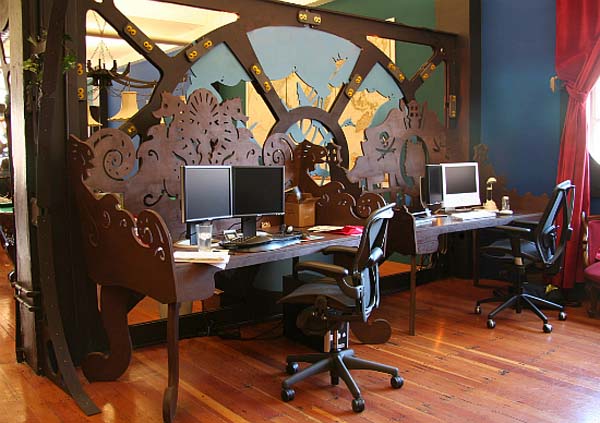This photograph captures an intricately designed office space, featuring two dual-monitor computer stations arranged on an elaborate wooden desk. The desk is adorned with ornate carvings of seahorses, seashells, and pirate flags, contributing to its unique nautical theme. Each computer station has a black mesh office chair equipped with lumbar support, armrests, and wheels. The floor is composed of amber wooden planks that complement the rich wooden features of the desk. Behind the desk, a matching privacy screen can be seen, which also follows the nautical motif. The walls of the room are predominantly blue, with glimpses of a green wall visible in an adjacent area through the openings in the privacy screen. On the right edge of the image, a red curtain partially covers a window, allowing light to stream into the room. This thoughtfully decorated space blends functionality with artistic detail, creating a distinctive and inviting atmosphere.